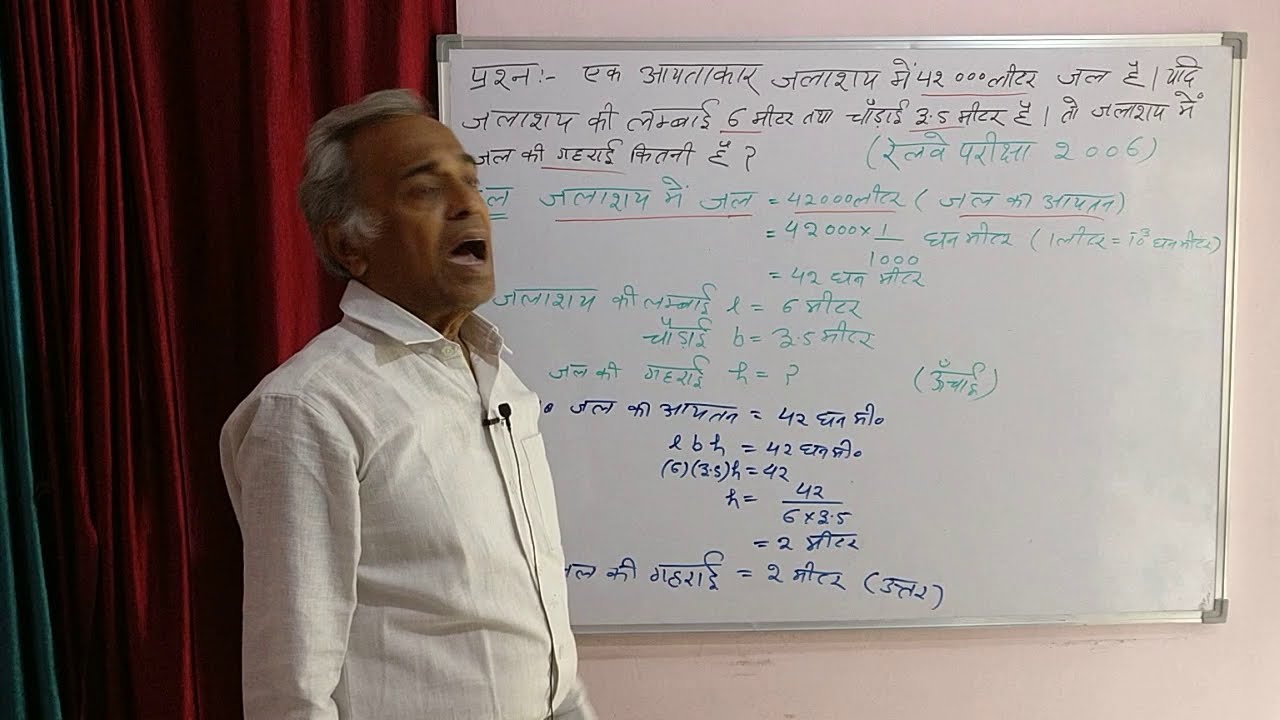In this image, a South Asian man, possibly in his 70s, stands slightly left of center. He is shown in a half-profile facing right, with his mouth open as if he is speaking. He is dressed in a full-sleeve white shirt and has a microphone clipped to its front. The man has short gray hair, black eyebrows, and a dark complexion. He is clean-shaven. Behind him on the left, a red curtain with a shiny gloss hangs down, and further to the corner, there are green curtains with a similar glossy texture. 

To the man's right is a large dry erase board against an off-white wall. The board is encased in a silver frame and filled with mathematical equations and text written in Hindi, using black, green, and dark blue markers. The board and the mathematical notations dominate the right side of the image, suggesting an educational setting, possibly a classroom, where the man appears to be giving a lecture on math. The colors in the image include red, green, white, brown, gray, black, blue, tan, and peach.